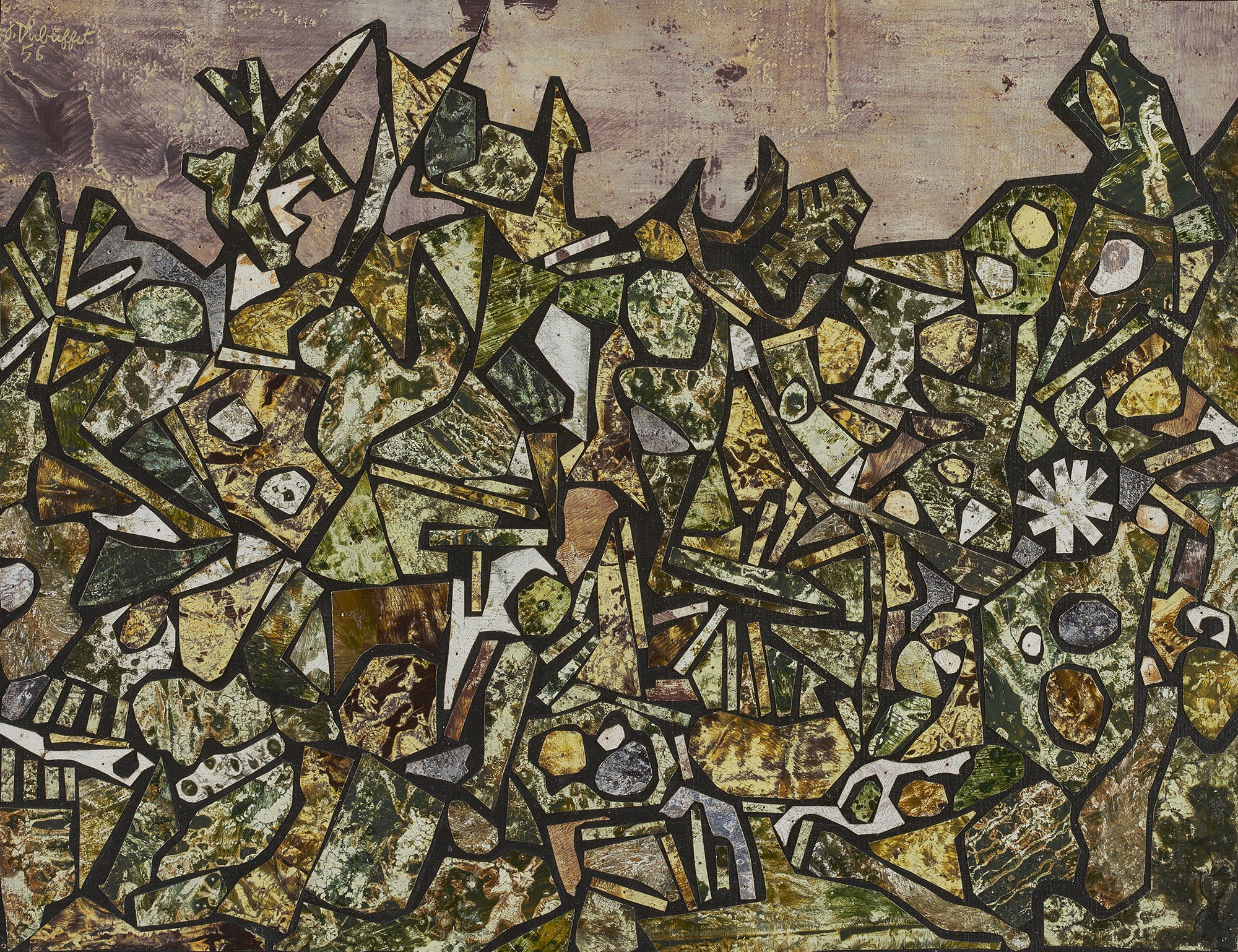The image depicts an abstract piece of artwork featuring a chaotic collection of geometric shapes, primarily in darker hues of green, gold, purple, and fall colors, all outlined in black. The shapes, which include round and elongated forms, are arranged on a dark, purplish, and grayish background, creating a visually complex pattern reminiscent of stained glass. The non-symmetrical and asymmetrical arrangement suggests a dynamic scene, evoking the imagery of an ocean wave with its in-and-out and up-and-down movement. At the same time, the dense clustering of shapes gives the impression of a chaotic battle or turmoil, with the shapes appearing to collapse in on one another. White and black spots interspersed throughout add to the contrast and depth, and although specific figures or scenes are indistinguishable, the overall effect is visually intriguing and artistically pleasing. There's also a section of the background that features a brownish tint at the top, adding to the complexity of the artwork.